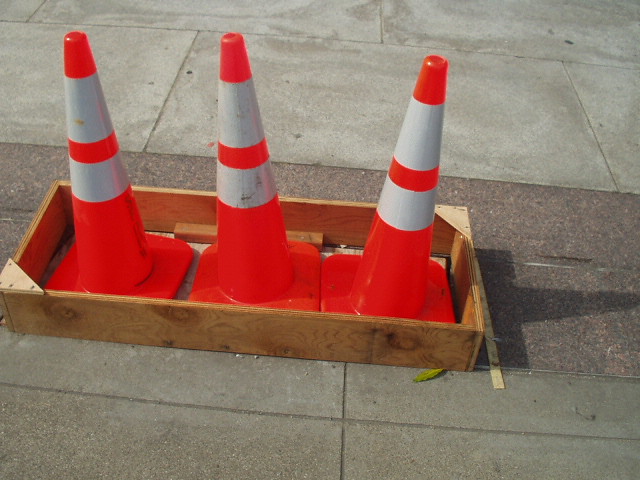This photograph, taken outdoors in daylight, depicts three bright orange traffic cones with two white reflective stripes each, neatly lined up in a light-colored, low-sided plywood box. The wooden box, made of four pieces of wood with wooden brackets on two corners, rests on a gray cement sidewalk. The sidewalk features a tile-like pattern with darker lines and a slightly mottled, darker area in the center. The cones, with their tall, skinny triangular shapes and rounded square bases, cast shadows on the concrete. A green leaf lies beside the box, adding a touch of nature to the urban scene. The overall setting is bathed in sunlight, highlighting details such as the cones' fluorescent shine and the box's smooth surface.